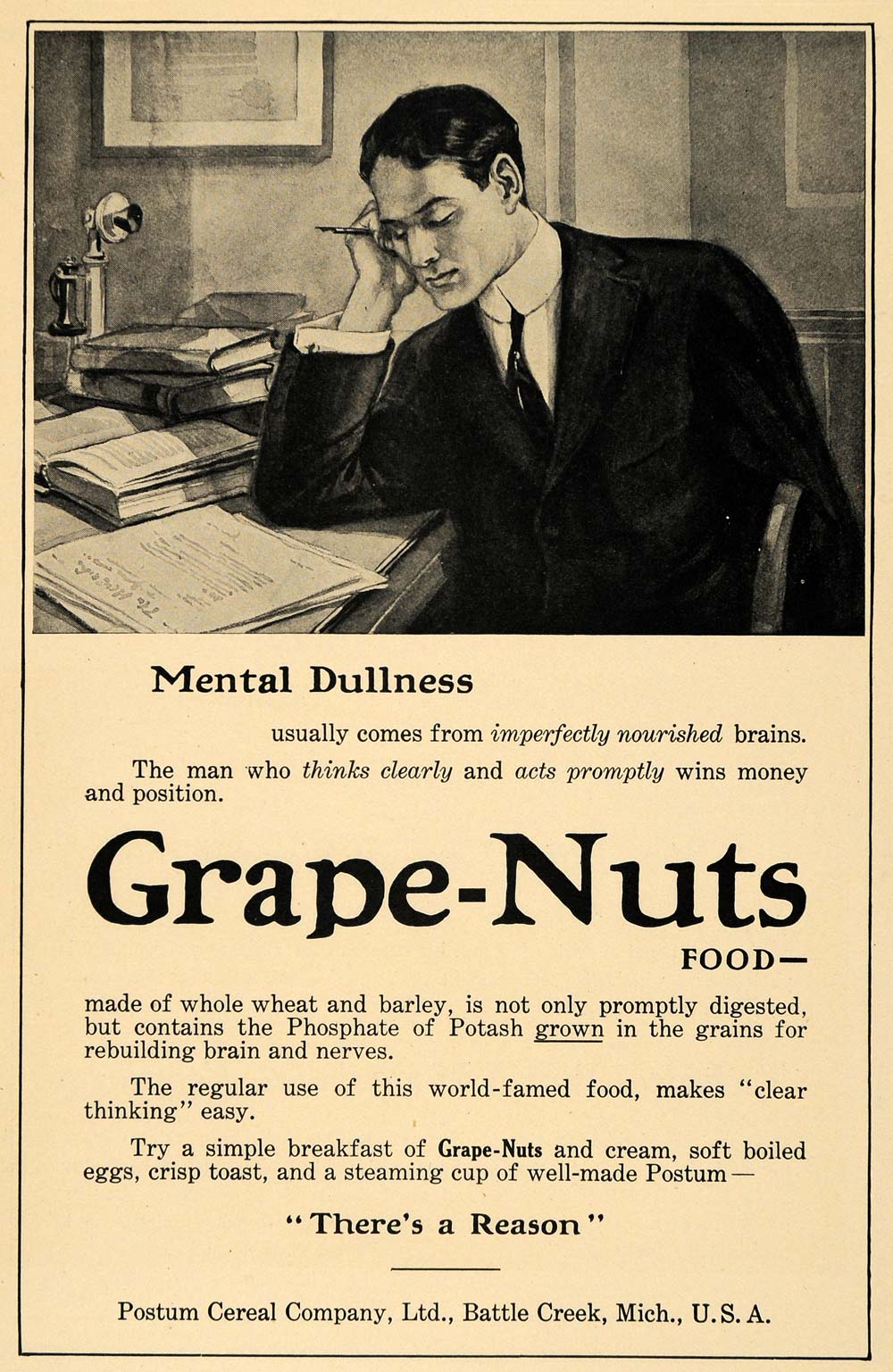The image is an intricately detailed, old advertisement for Grape Nuts cereal, possibly from a magazine. It features a black-and-white illustration of a young man, likely an office worker or lawyer, dressed in a suit with a high collar and tie. He is depicted dozing off at a cluttered desk, resting his head on his hand. The desk is laden with papers, open books, and a candlestick phone, while the background includes framed artwork and part of a panel door.

The advertisement text is quite extensive and emphasizes the benefits of Grape Nuts for mental acuity. Below the image, it states: "Mental dullness usually comes from imperfectly nourished brains. The man who thinks clearly and acts promptly wins money and position." It goes on to highlight that Grape Nuts, made from whole wheat and barley, contains phosphate of potash grown in the grains, which is essential for rebuilding brains and nerves. The ad claims that regular consumption of this celebrated food makes clear thinking easy. It suggests a breakfast combination of Grape Nuts and cream, soft-boiled eggs, crisp toast, and a steaming cup of well-made Postum. The tagline concludes with the slogan in quotes, "There's a reason," attributed to the Postum Cereal Company, Battle Creek, Michigan, USA.